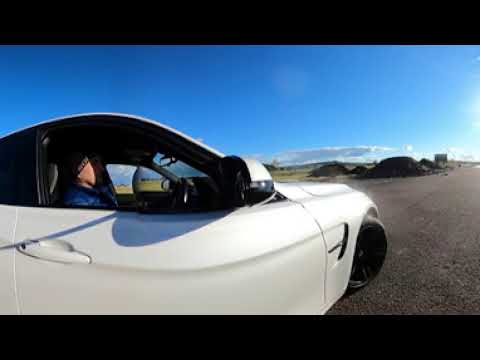The photo depicts an outdoor scene focused on the right side of a white car, potentially a sports car, sedan, hatchback, or coupe. The viewpoint shows the front portion and the front doors of the vehicle. Inside the car, on the right side, there's a male occupant, likely the driver, indicating the car might be in a country where vehicles have right-hand drive. He is a white male, wearing a black hat and a blue jacket. Only his upper body is visible from the neck to the shoulder. The car seems to be driving on an open gravel road without marked lanes. The background reveals green grass, rocky outcrops, and hills or mounds of dirt. The sky is predominantly clear and blue, with a few white clouds lingering on the horizon, contrasting with the otherwise bright, sunny day.